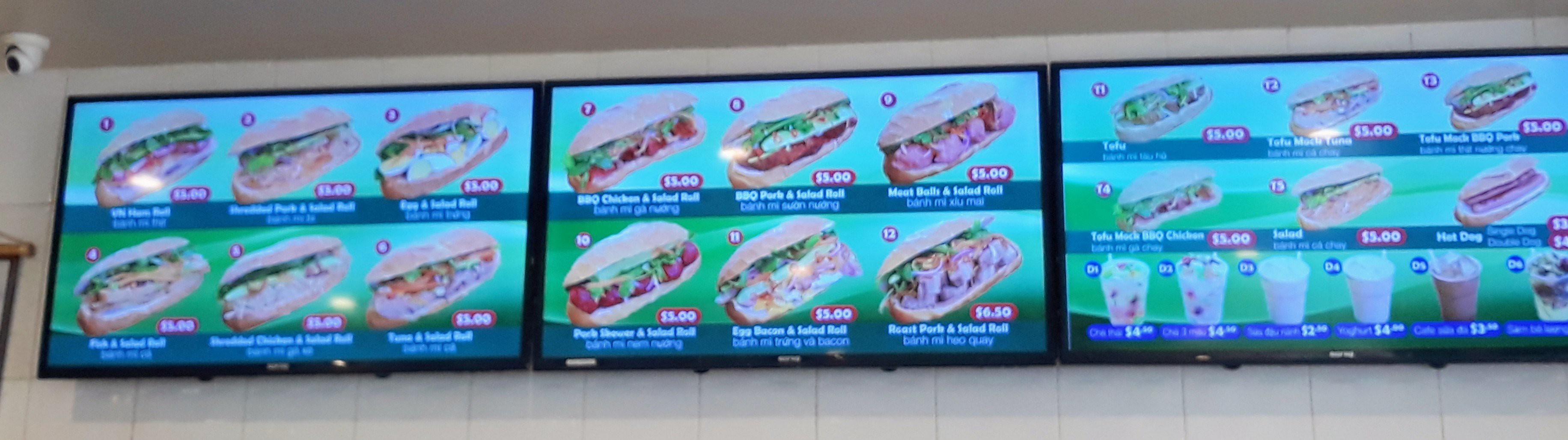A brightly lit menu mounted on a white industrial tile wall displays offerings from a submarine sandwich shop. The menu is organized into three rectangular panels. 

The first two panels are each divided horizontally into two sections, with every section featuring three submarine sandwiches against a blue background. The names of the sandwiches are written in white text over a blue banner, and the prices are clearly indicated in white text on a red banner below each name.

The third panel is divided into three sections: the top two sections showcasing another set of three submarine sandwiches each, while the bottom section features an assortment of six beverages. 

Each sandwich image is vibrant and appetizing, promising a delicious meal, while the drink section adds refreshing options to the mix. The clean, tile-mount background lends an industrial feel to the fast-food joint’s visual presentation.